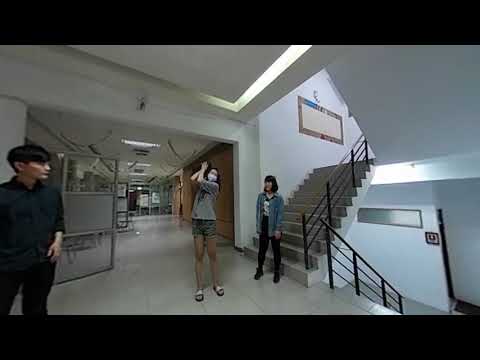The image depicts three students, likely of East Asian descent, inside a dormitory or student congregation area with white or eggshell-colored walls and grayish flooring. A stairwell is visible on the right, with both ascending and descending staircases. The scene is slightly distorted, making the individuals appear taller and thinner than usual. 

At the center, a woman wearing a gray, long-sleeved shirt, cut-off jeans (or possibly green shorts), and sandals stands, her hands raised above her head as though she's in the motion of swinging a golf club or preparing to throw something. She is also wearing a white mask. To her right, at the base of the upward staircase, is another woman dressed in black jeans, a denim jacket, and a black t-shirt with a white emblem. On her left stands a gentleman clad in all-black attire, including a long-sleeved shirt. 

Further into the background, there are white walls adorned with recessed fluorescent lighting and an entranceway that appears to lead into another section of the building, with visible windows and doors.